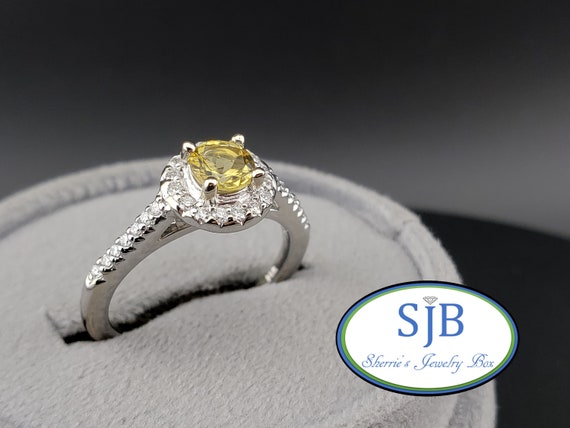This close-up advertising photograph showcases a dainty, platinum engagement ring with a thin band and four prongs securing a striking yellow diamond at its center. Flanking the vibrant center stone are small, shimmering diamonds that extend equally on both sides of the band. The ring sits elegantly within a gray felt ring box, set against a dark, black background. In the lower right corner of the image, the logo "SJB Sherry's Jewelry Box" is prominently displayed, featuring blue letters underneath a diamond icon, highlighting the ring's luxurious origin. The ring is angled to accentuate its intricate details and sparkling brilliance, making it the focal point of the image.